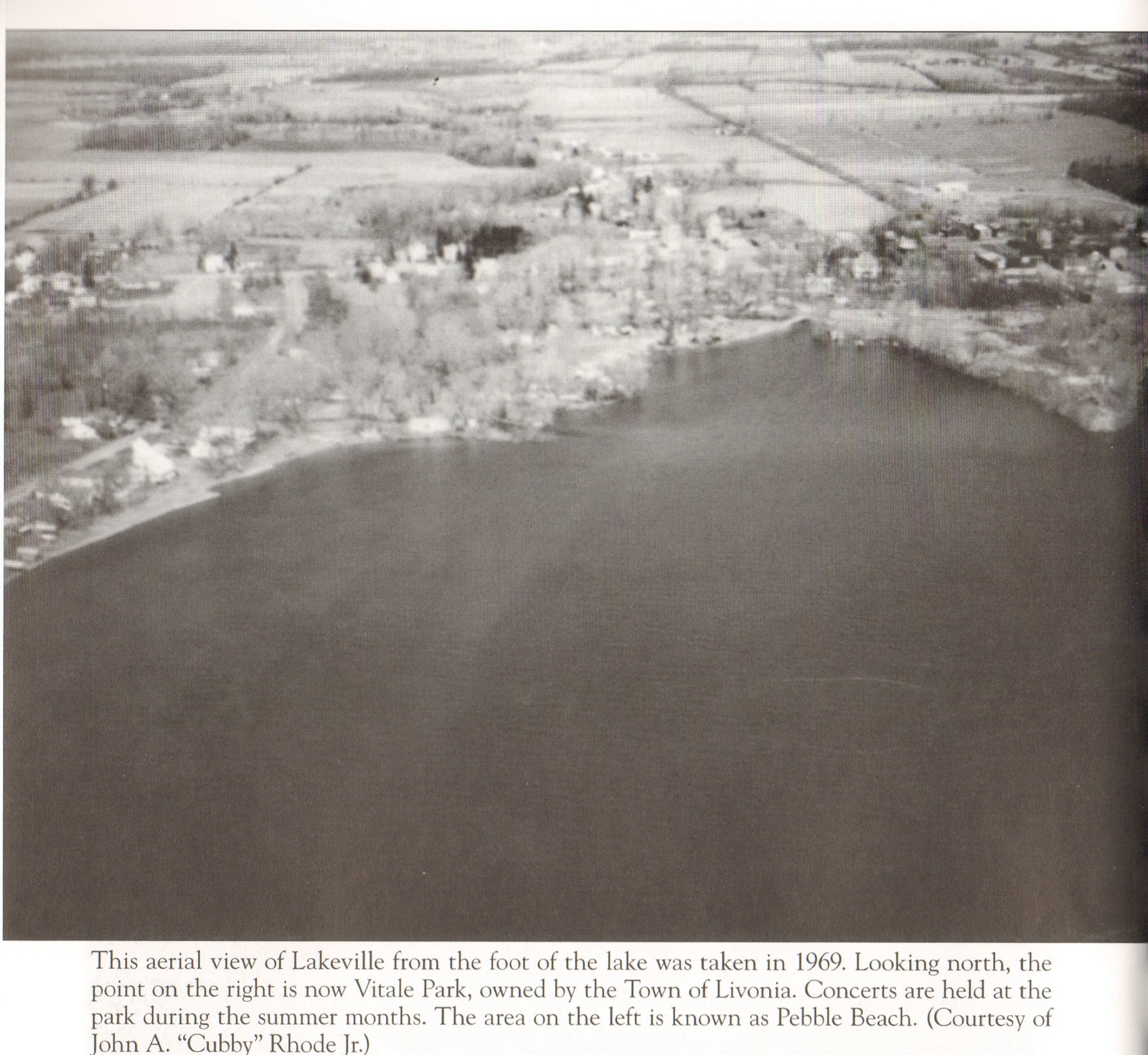This is an old, black and white aerial photo of Lakeville taken in 1969, looking north. The lake is predominantly at the bottom of the image, with the surrounding land featuring trees, pastures, fields, and a few buildings. To the right of the lake is a point that has since become Vital Park, now owned by the town of Livonia, where summer concerts are held. On the left side of the lake, there's an area known as Pebble Beach, credited to John A. "Cubby" Rowe Jr. The image is somewhat fuzzy and blurred, but the descriptive text at the bottom offers clear context and historical insight into the scene depicted.